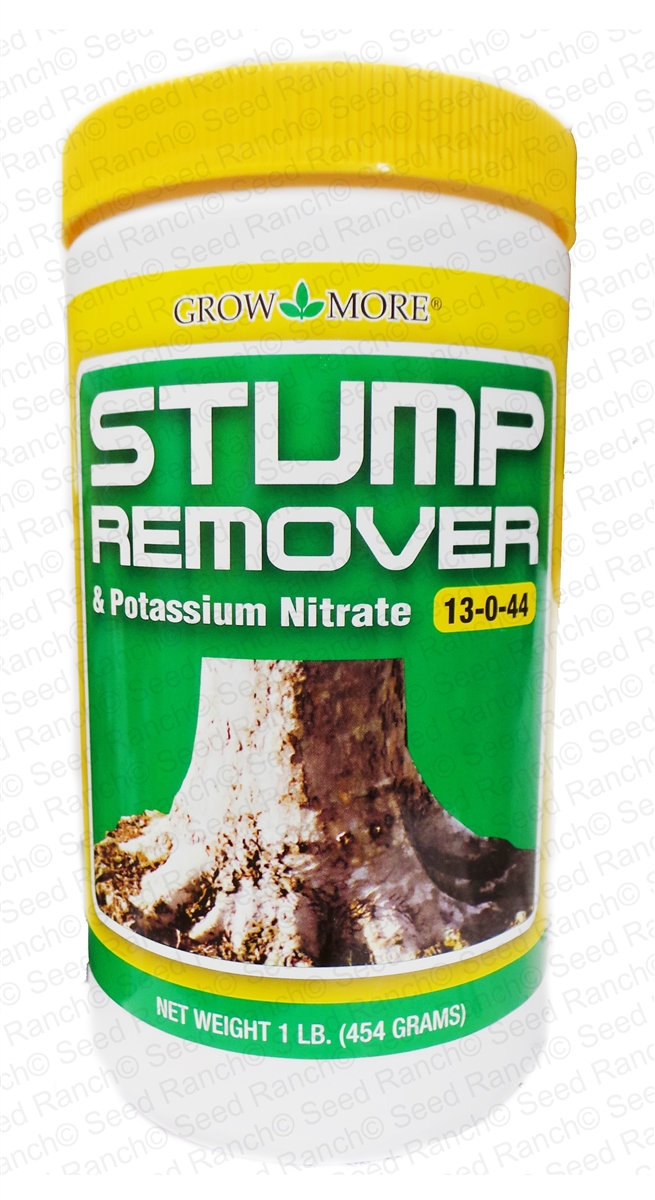The image features a detailed, color photograph in portrait orientation showcasing a cylindrical, white plastic jar of stump remover. The jar is fitted with a yellow screw-on lid. The upper portion of the jar displays a yellow label stripe, which prominently features the words "Grow More" in black text flanked by a leaf logo. Below this, the main portion of the label has a green background with "STUMP REMOVER" printed in bold, white capital letters. Underneath, it reads "and potassium nitrate," also in white text. On the right side of the label is the numerical formula "13-0-44" in yellow. The lower part of the label features an image of a tree stump, whose bark has been partially peeled away, revealing a yellow-brown substance on the surface. At the very bottom, within a green border, the label reads "Net Weight 1 Pound (454 grams)" in white text. The style of the product photography is realistic and detailed, showcasing the jar effectively. A gray watermark diagonally spans the image with the text "Seed Ranch."